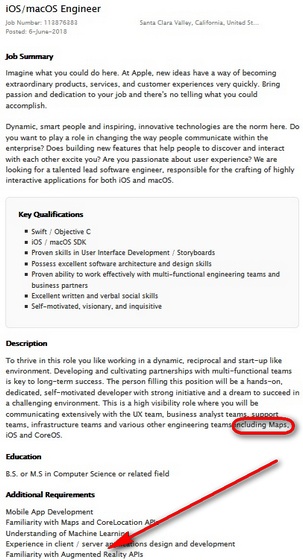**Caption:**

The image appears to be a screenshot of a resume for an "iOS/Mac OS Engineer." At the top, the title is prominently displayed with the job number and a posted date of June 6, 2018, alongside the location in Santa Clara Valley, California. The job summary section begins with an inspiring statement: "Imagine what you could do here at Apple. New ideas have a way of becoming extraordinary products, services, and customer experiences very quickly. Bring passion and dedication to your job, and there's no telling what you could accomplish. Dynamic, smart people, and inspiring innovative technologies are the norm here." The summary invites potential candidates to play a role in transforming internal communications by building new features that enhance user interactions. The position seeks a talented lead software engineer skilled in developing highly interactive applications for both iOS and Mac OS.

Additionally, a section of key qualifications and a detailed description is visible. Notably, the word "maps" is circled in red, with an arrow pointing to the bottom of the screen under the "Additional Requirements" section, specifically highlighting the need for "familiarity with augmented reality APIs."